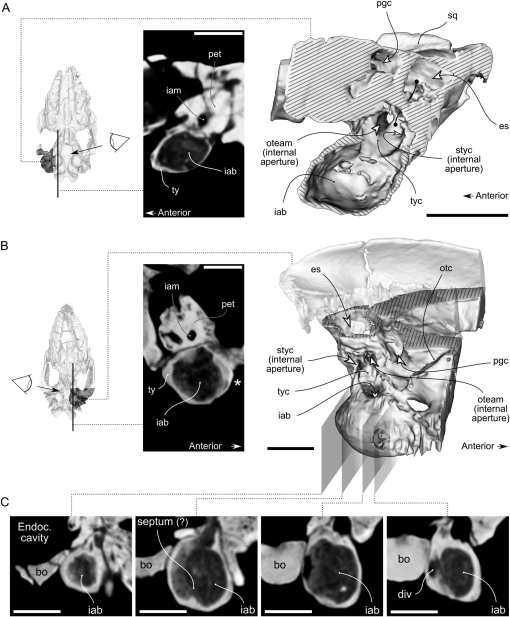The image showcases a comprehensive medical study, comprising a series of black-and-white diagnostic displays and scientific diagrams focused on the anatomy of a human nose, specifically detailing the endocavity and septum. The structured layout is organized into three labeled sections – A, B, and C.

Section A presents three distinct images: a preliminary anatomical drawing, a corresponding black-and-white photograph, and a detailed illustration with various parts labeled by arrows and annotations, such as 'anterior' and 'internal aperture'. 

Section B also contains three images. It begins with a diagram, followed by a contextual black-and-white photograph, and concludes with a detailed anatomical diagram indicating the precise location of various features within the body, highlighting terms like 'STYC internal aperture' and 'PGC'.

Section C includes four x-ray-style photographs. These images meticulously display different views and magnifications of the endocrine cavity and septum, alongside labels that might contain abbreviations or identifiers such as 'BOIAB'.

Overall, this intricate assemblage of drawings, photographs, and x-rays offers an in-depth visual analysis of nasal cavity structures, emphasizing the septum and internal apertures.